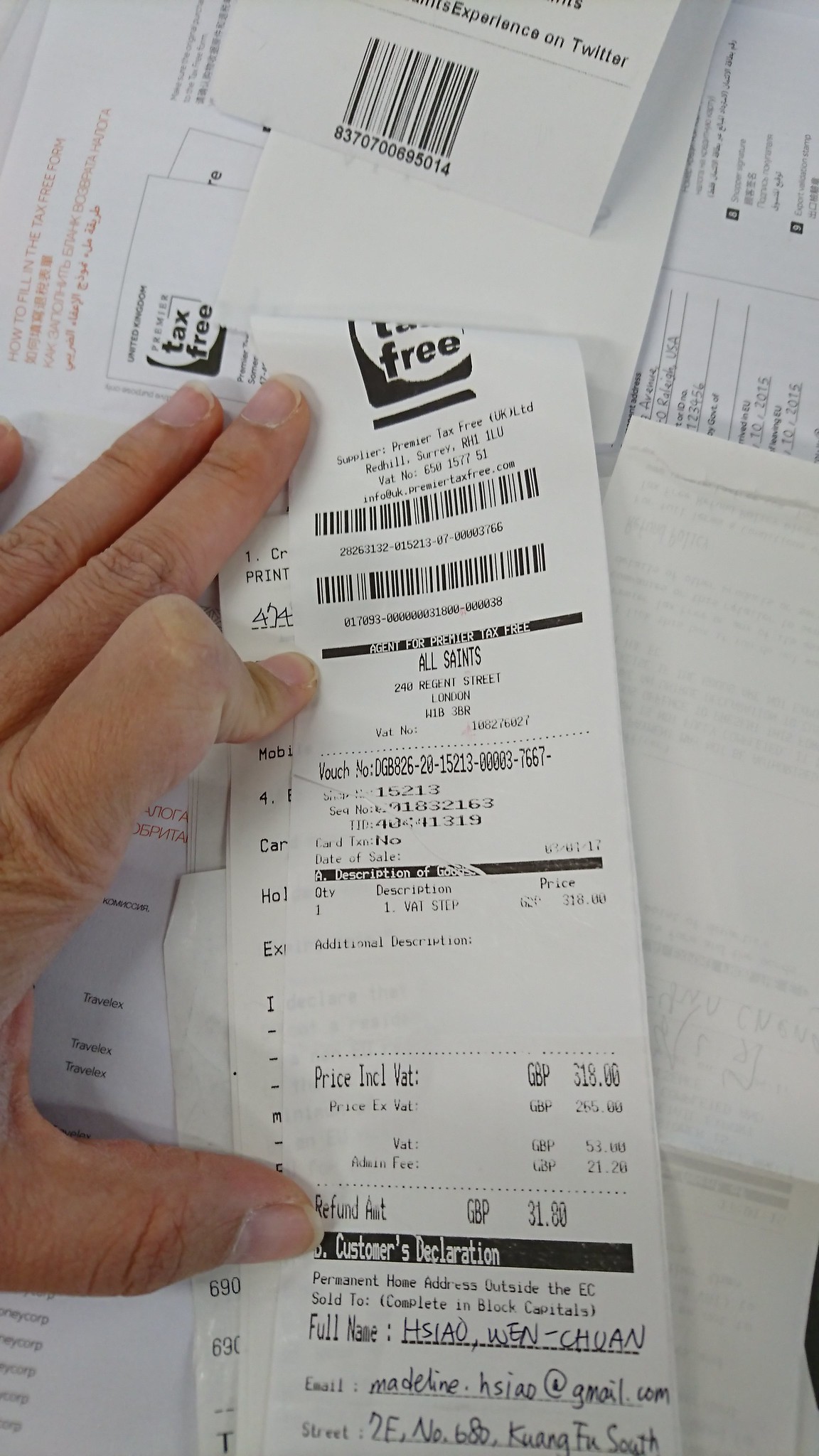In the image, a slightly tanned, dry-skinned left hand, with an index finger bent in a peculiar shape, holds down a white receipt. The hand, seemingly hyper-mobile, is positioned with fingers near the top and the thumb near the bottom, preventing the receipt from curling up. The receipt, from a store called All Saints, shows a purchase amount of £318 GBP. The top of the receipt has two barcodes and states "tax-free." It also includes detailed information about the business location and address. A customer's declaration section at the bottom contains handwritten details: the customer's name is Wen Chuan Hoi Sao, their email is madeleine.sae@gmail.com, but the street address is partially unreadable. Surrounding the receipt are numerous other white pieces of paper, including what appear to be additional receipts, business documents, and tax papers, creating a cluttered desk covered in paperwork.